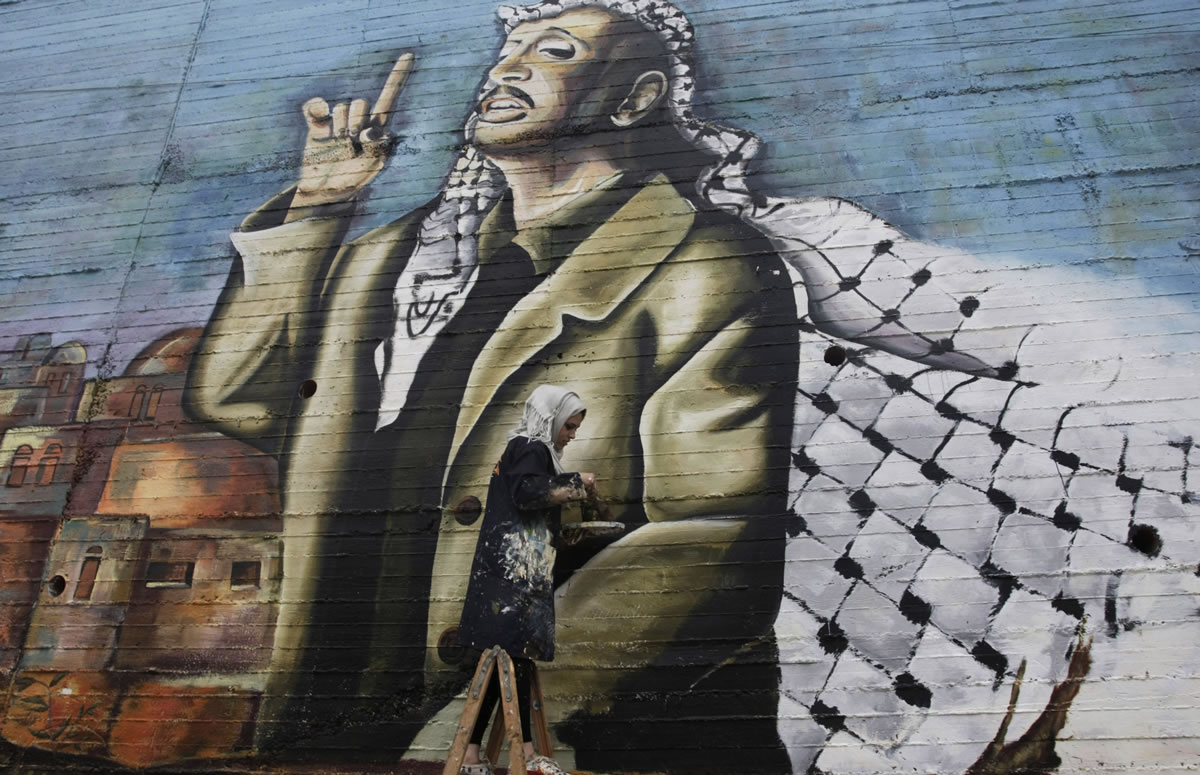This horizontal, rectangular photo captures a large, outdoor mural, occupying the majority of the frame. The mural, painted against a backdrop of light blue, prominently features a striking image of Yasser Arafat in the middle. Arafat, identifiable by his iconic, exaggerated white checkered keffiyeh, which extends dramatically across three-quarters of the mural, is depicted wearing a tan overcoat over a black shirt. His right arm is bent at the elbow, pointing a finger upward toward the sky. To the left of Arafat's elbow, the mural includes stylized, dilapidated houses, emphasizing the setting.

The mural appears to be painted on a wooden surface, as indicated by horizontal slats in the background. In the foreground, an Arab woman artist, dressed in a black, paint-splattered coat and a white hijab, is seen standing on a ladder. She is actively engaged in her work, dipping her brush into white paint and adding finishing highlights to Arafat's coat. The scene evokes themes of Palestinian identity and resilience.